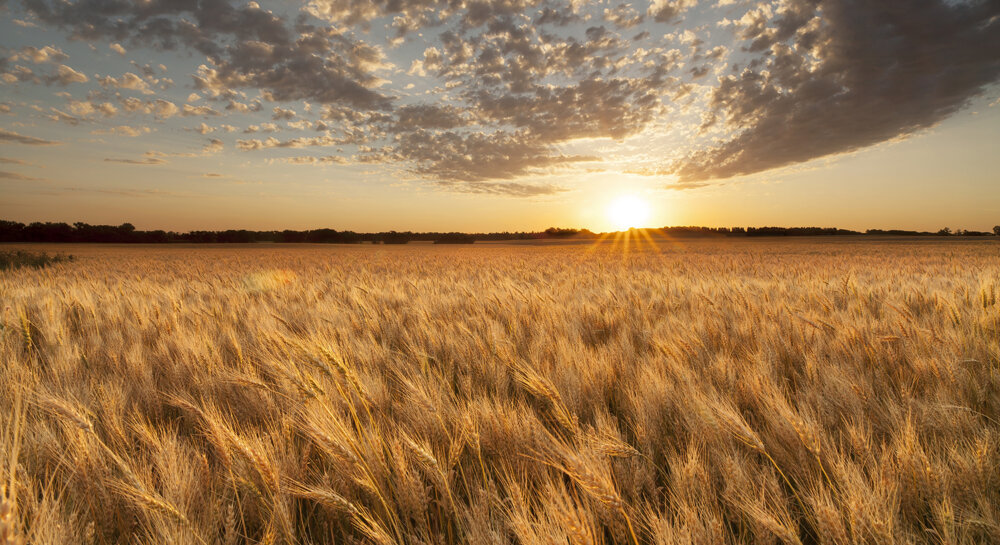The image portrays a serene wheat field during the early morning or at sunset, with the sun just above the horizon, exuding a warm, golden glow that bathes the scene in hues of orange and yellow. The expansive field is a sea of light brown, wispy wheat tops, gently curved, possibly indicating a light breeze. The horizon, marked by a dark line of trees, remains untouched by human presence, emphasizing the natural tranquility of the landscape. The sky is a gradient of orange transitioning into deeper blue, dotted with numerous clouds—some large and prominent, others smaller nimbus clouds scattered throughout. Near the left center of the image, a darker, non-wheat element adds subtle contrast. The overall palette includes grays, yellows, browns, blues, and touches of white from the clouds, evoking a peaceful and timeless rural scene.